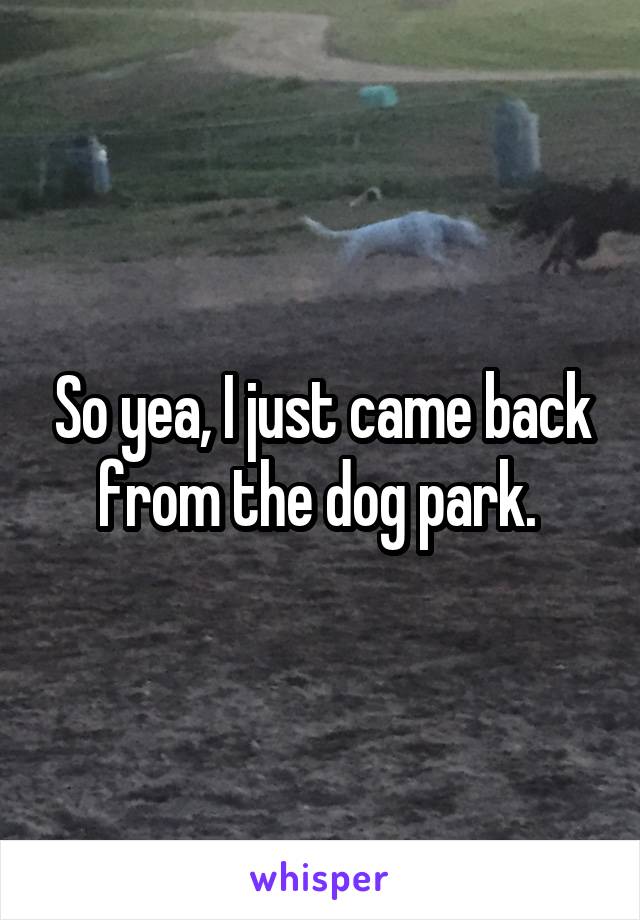In this grainy, low-resolution photograph predominantly featuring a dusty, sandy field, the bottom two-thirds to three-quarters of the image is filled with dirt, transitioning to a strip of grassy area at the upper portion where a dirt road or trail is visible. The scene captures lively motion with visible blurriness, as a white dog in full view to the right chases after one, possibly two darker-colored dogs, whose partial figures are disappearing off the screen. The setting resembles a somewhat neglected fenced farm or yard, dotted with a couple of indistinguishable cylindrical objects and a strange green item resembling a mailbox without a pole. Central to the image, in large white text, is the caption, "So yeah, I just came back from the dog park," suggesting a casual, playful context. Beneath the photo, on a white band, is the watermark "Whisper," hinting at the platform where the image was shared. The image employs a palette of mostly brown, beige, and green hues, emphasizing the earthy, rustic setting.